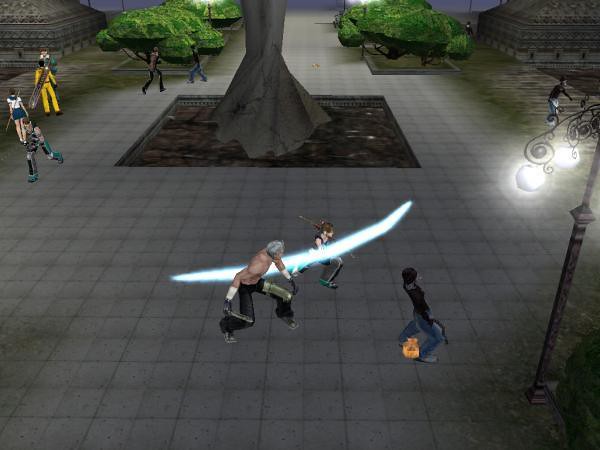In this dynamic video game scene, a large, muscular man with gray hair, wearing black pants and white wristbands, charges forward shirtless. Beside him, a younger woman in a black tank top runs with a focused expression while gripping a long gun. A pulsating, luminous beam stretches between them, illuminating their determined stride.

In the mid-ground, a conspicuous man dressed in black appears to be the target, clutching an orange bag as he also sprints forward. The action unfolds in a bustling courtyard dominated by a colossal tree, its trunk encased in sculpted bark and surrounded by interlocking brickwork. Towering evergreens form a natural backdrop on either side of a walkway that cuts through the scene.

To the right, a building comes into view, adding an urban element, while another man is seen walking nearby. To the left, a street lamp with a steel finish casts light over a crowd of people in various postures; some stand idle while others move. The ensemble is a mix of shades of yellow, black, and tan attire. Among them, a woman dressed in shorts and a white T-shirt is distinctly visible.